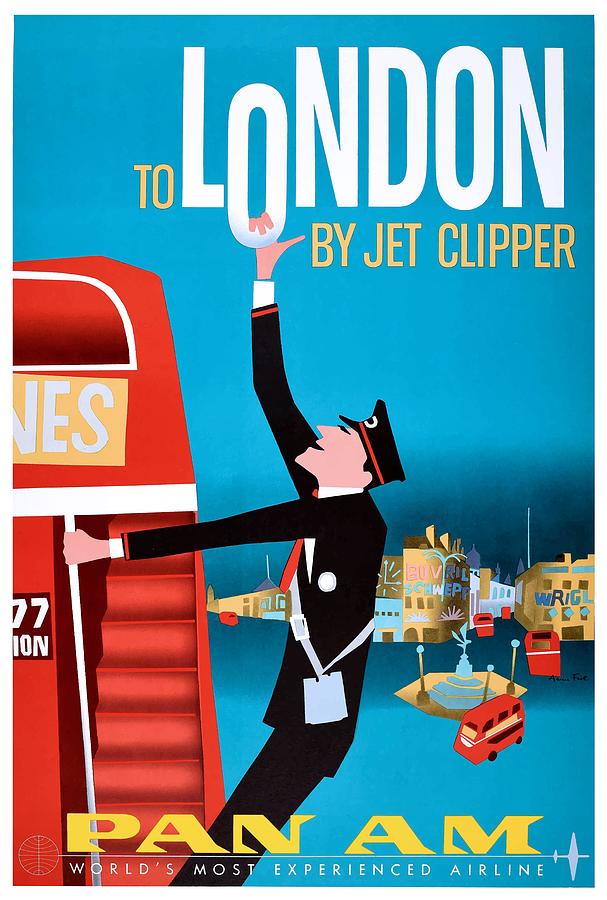This is a vertically oriented, full-color vintage poster advertising Pan Am flights to London. The background is a blue sky, and the top prominently features the word "London" in large white letters. The 'O' in "London" is cleverly designed with a man's hand gripping it, giving the illusion that it is being pulled down. This man, who appears to be a conductor or a postman, is dressed in a blue uniform, white shirt, red tie, and a blue cap with a white pin on his left breast. He is hanging onto the 'O' while climbing a red double-decker bus. To the left, there are smaller graphic elements depicting a double-decker bus in the city. To the upper left in yellow letters, it says "Two" and beneath it "By Jet Clipper." At the bottom of the poster, the Pan Am logo is displayed with the slogan "World's Most Experienced Airline" written in white letters.